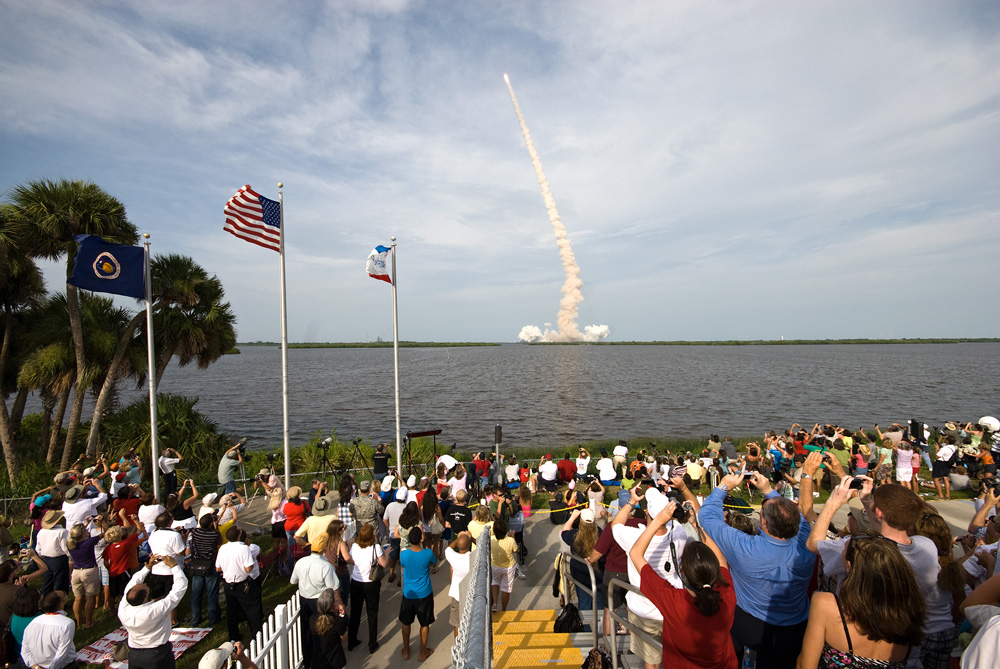This color daylight photograph captures a large group of people gathered in a viewing area, all with their backs turned to us, holding up cameras and phones. They are witnessing the launch of a space rocket. On the left, there are three flagpoles displaying a blue flag with a circular planetary logo, a red, white, and blue striped flag, and the American flag in the center. In the background, there's a lush green area with trees, which transitions into a vast flat body of water leading to a distant shore with low-lying greenery. Dominating the sky is a dramatic scene of a rocket launch: a massive plume of gray and white smoke at the bottom that extends into a long vapor trail reaching upward. The bright tip of the rocket burns vividly at the top of this trail, piercing through the slightly cloudy sky. The scenic mixture of terrestrial and celestial elements underscores the monumental human endeavor taking place.